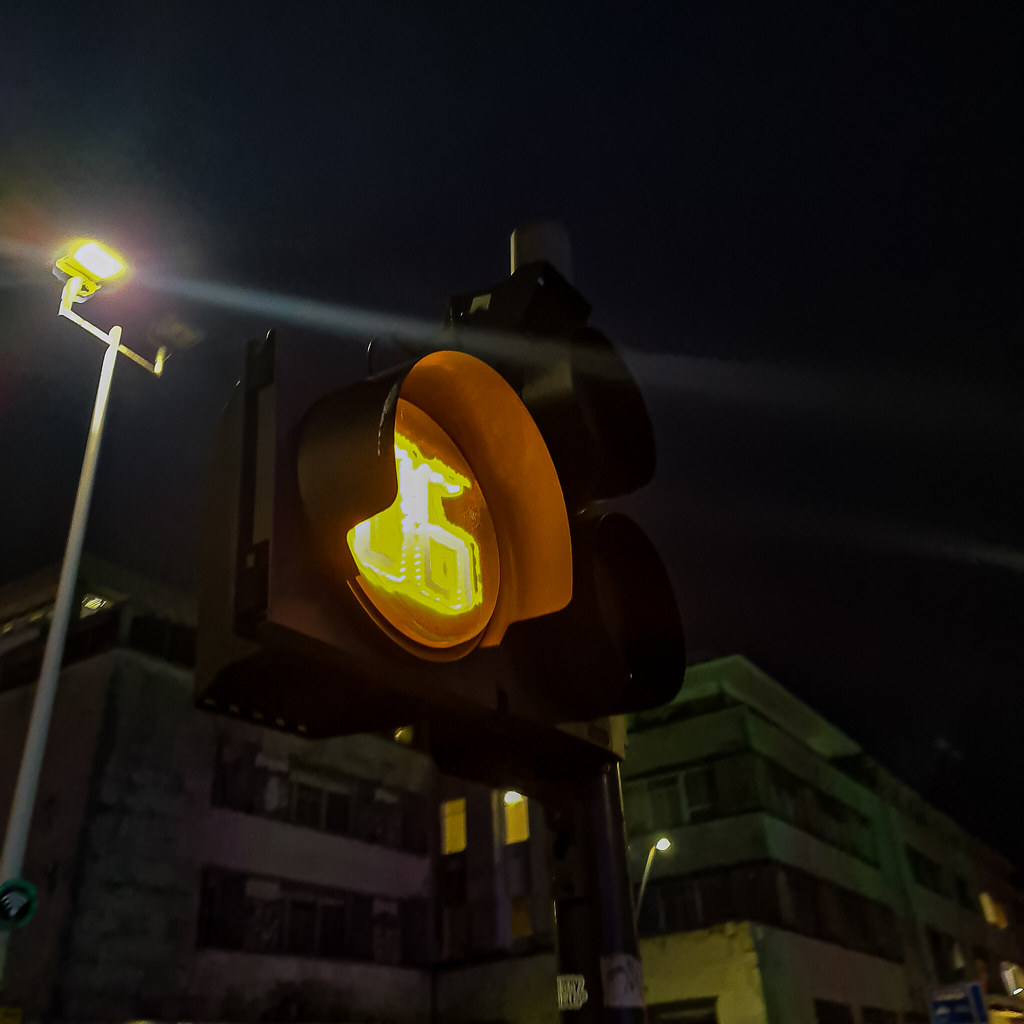This captivating night-time photograph, set in an urban environment, showcases an intriguing street scene. Dominating the foreground is an electronic street sign, radiating a warm, inviting glow with its bright yellow and gold lights. The sign, which displays the number "06," is mounted on a dark-colored metal pole, adding to the industrial yet charming city atmosphere.

Adjacent to this, a tall streetlight stands proudly on a sleek silver metal pole, casting a soft yellow light that gently illuminates the surrounding area. An ethereal shaft of white light bisects the image, adding an element of mystique.

In the backdrop, the cityscape is framed by several multi-story buildings, their light-colored facades largely shrouded in darkness. Only a few windows emit a faint glow, hinting at the life within. Additional streetlights are faintly visible in the distance, further enriching this nocturnal urban tableau.